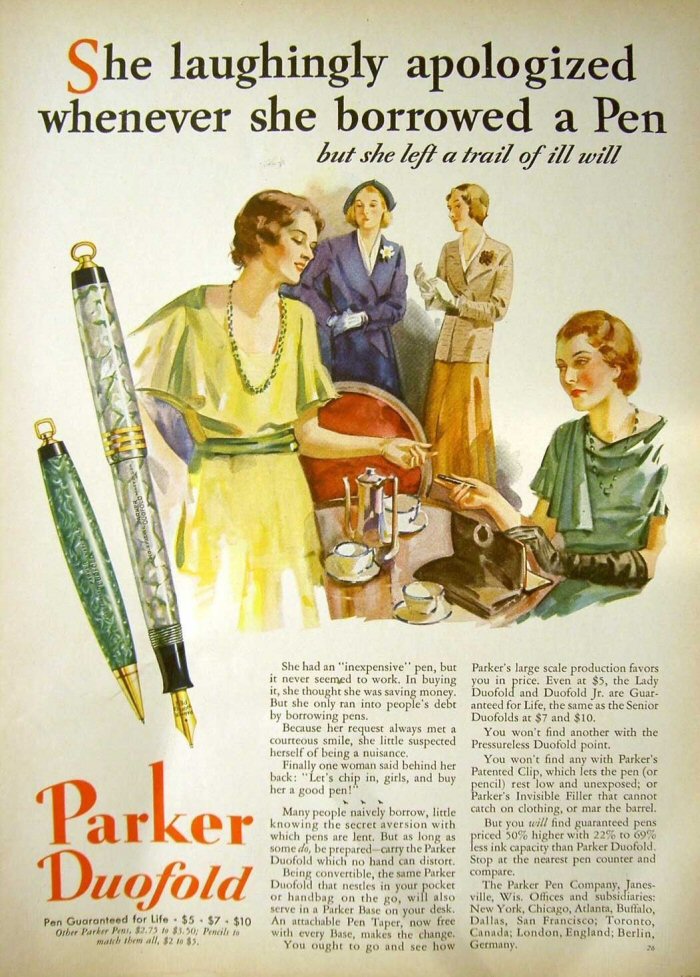This vintage magazine advertisement for Parker Duofold pens, set against a light gray background, showcases an elegant scene of four women dressed in 1930s or 1940s fashion. The ad captures a moment where one woman, seated and dressed in a fancy green dress with black gloves, reaches into her purse to hand a pen to another woman standing before her. The woman receiving the pen wears a yellow dress with a long necklace and green belt. In the background, two more women stand poised in fashionable suits—one in a blue suit with white gloves and a matching hat, and the other in a tan suit with an orange skirt. At the top, bold text reads, "She laughingly apologized whenever she borrowed a pen, but she left a trail of ill will." In the left margin, two intricately designed fountain pens are displayed, one mostly marble green and the other predominantly white. Below the pens, vibrant red text announces, "Parker Duofold," followed by a guarantee for life, stating prices of $5, $7, and $10. A detailed narrative extols the virtues of Parker Duofold pens, emphasizing their reliability, the unique pressureless point, and patented clip design, aiming to encourage potential customers to compare and choose Parker pens, available at multiple locations globally. In the bottom right corner, the number 26 is subtly noted.